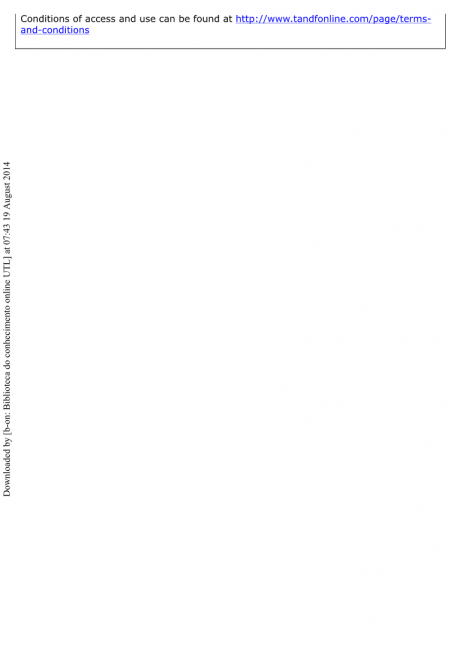This image appears to depict a partial screenshot of a webpage, with notable text details. The central portion features a blank or obscured area, making it difficult to identify the specific section of the site. On the left-hand side, there is a diagonal sentence in small black print that reads, "Downloaded by [illegible] at 07-4319 August 2014." The garbled text underneath includes "biblical" and other undecipherable words.

At the top of the image, a long rectangular box presents text in a larger and more readable font. It states, "Conditions of access and use can be found at," followed by repeated lines of the URL: "http://www.tandfonline.com www.tandfonline.com www.tandfonline.com www.tandfonline.com www.tandfonline.com www.tandfonline.com www.tandonline.com."